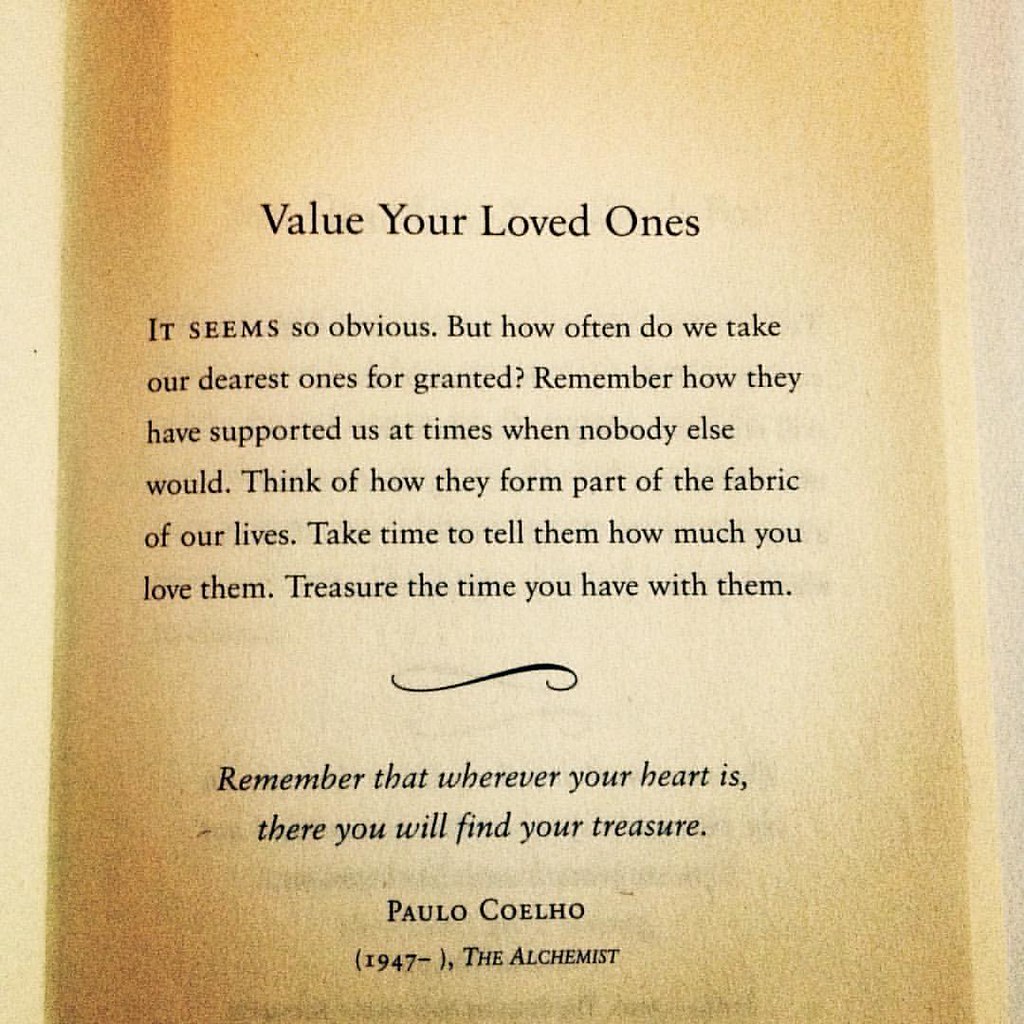The image is a tightly zoomed-in photograph of a page, likely from an old book or pamphlet. The page has a weathered, parchment-like appearance, with hues ranging from light brown to dark brown, especially at the edges. A prominent black text at the top reads, "Value Your Loved Ones." Below this title, in smaller black print, the text elaborates: "It seems so obvious, but how often do we take our dearest ones for granted? Remember how they have supported us at times when no one else would. Think of how they form part of the fabric of our lives. Take time to tell them how much you love them. Treasure the time you have with them." 

Following this passage is a curved divider, resembling a fish hook. Beneath the divider, another quote appears in a different, handwritten-style font: "Remember that wherever your heart is, there you will find your treasure." This quote is attributed to Paolo Coelho, with the text "Paolo Coelho (1947 - )" indicating that he is still living. He is referred to as "the alchemist." The overall aesthetic of the page combines nostalgic and literary elements, accentuated by the aged, yellow-brown texture of the paper.